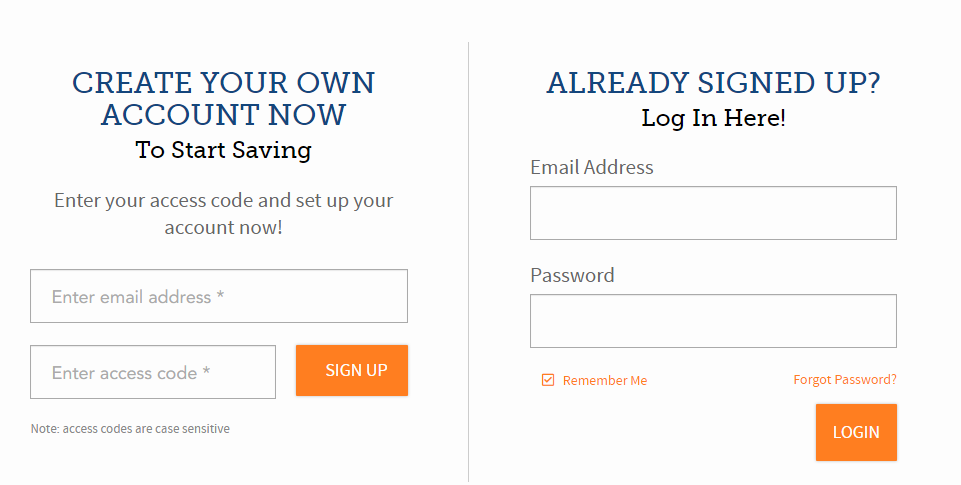Image Caption: 

The image displays a dual-section interface for account creation and login. The left section, dedicated to new users, prompts individuals to "Create Your Own Account Now to Start Saving." Users are instructed to enter their email address and an access code, noting the case sensitivity of the codes. A prominent orange "Sign Up" button facilitates the account creation process.

The right section caters to returning users with the header, "Already Signed Up? Login Here." This section provides fields for email address and password entry, alongside a "Remember Me" checkbox for convenience. Below these fields, there is a subtle orange "Forgot Your Password?" link for password retrieval. A large orange "Login" button completes the login process.

While the exact purpose of the account creation and saving is unclear, as some information appears to be missing, the page is intuitively designed for easy sign-up and login, denoted by the clear prompts and uniform orange action buttons.